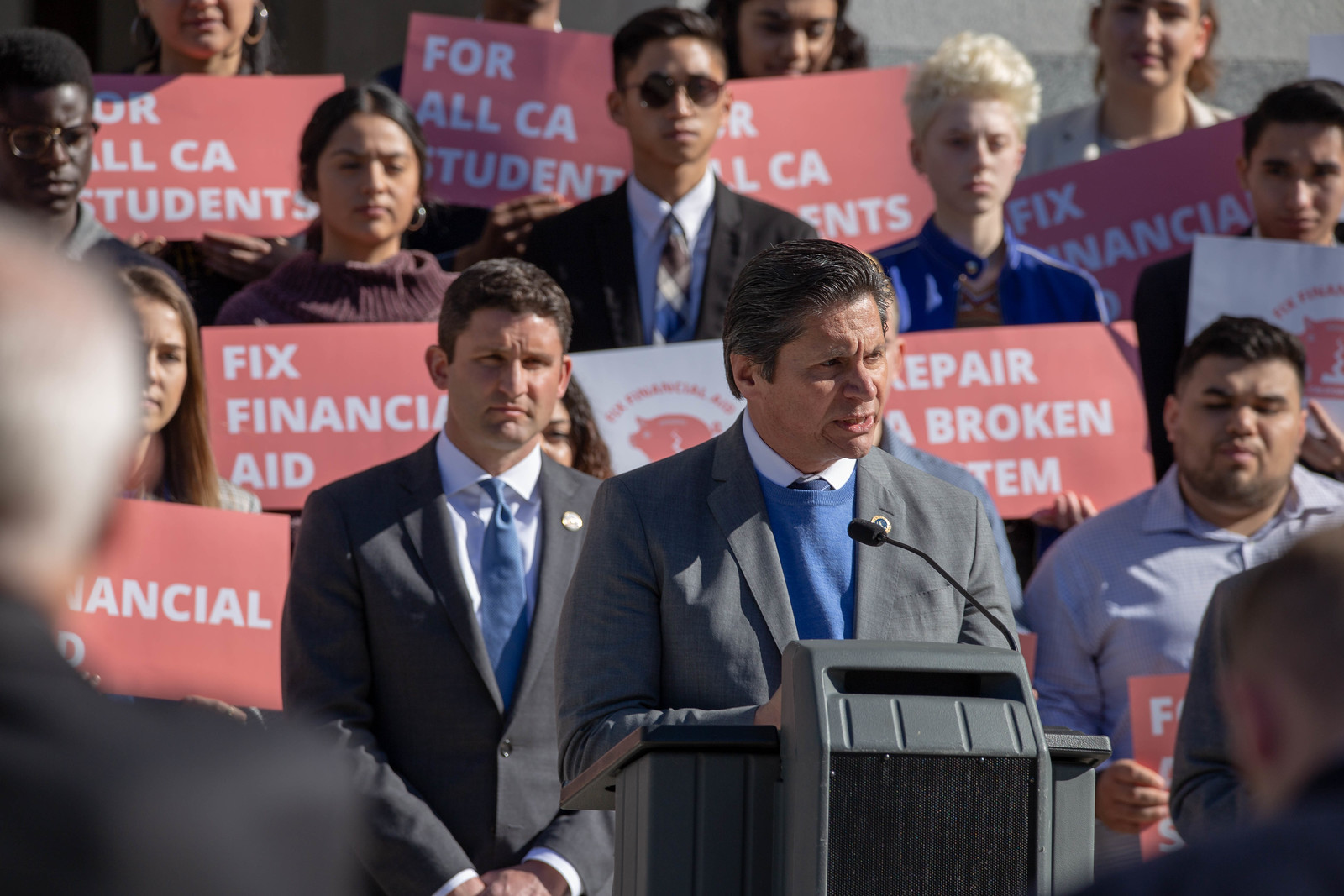In this photograph, a politician stands at a podium delivering a speech, with a microphone in front of him. He is clean-shaven and dressed in a grey suit jacket over a blue sweater, revealing a white dress shirt with a bit of his tie peeking out. Both he and another man behind him—also in a suit and tie—wear lapel pins. Behind them, a diverse group of young people holds up various placards displaying slogans such as "fix financial aid," "repair broken system," and other calls for reform. The crowd includes individuals of different cultures and genders. In the foreground, partially visible on the left and right, are two figures that appear to be security personnel, dressed in suits and facing the audience, adding a layer of formality and protection to the event. The scene is charged with a sense of urgency and collective demand for change.